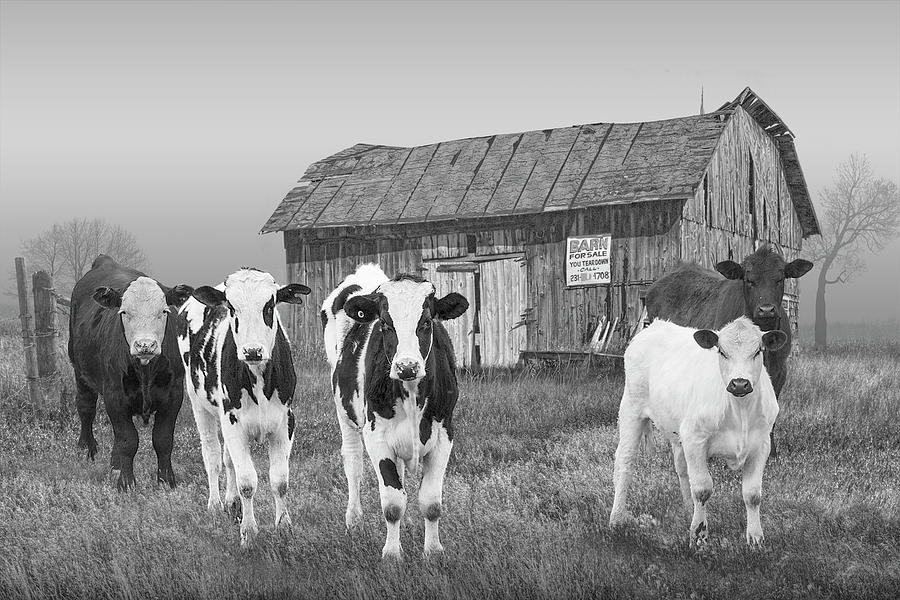In this black and white image, five cows are standing in a grassy field and all are looking directly at the photographer, creating a somewhat menacing impression. The cow on the far left is entirely white with distinctive black ears. Beside it are three white cows adorned with black spots. There is also a purely black cow, and one black cow with a strikingly white face. Behind them stands a dilapidated wooden barn, featuring visible holes and cracks in the roof and side panels. The barn has two white doors and bears a sign reading "Barn for sale" with additional, illegible text. Flanking the barn are two trees—one in the right-hand corner and another on the left side of the image. The scene is enveloped in a slight haze, adding to the nostalgic, rustic atmosphere.